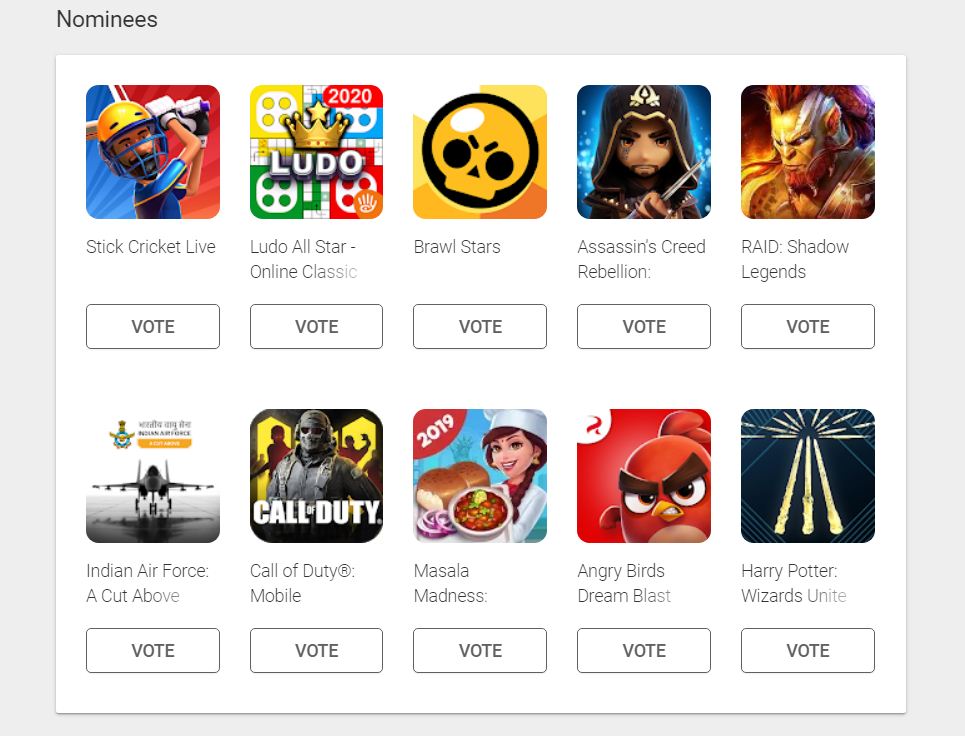This image depicts a screen featuring a voting interface for various game nominees. The background is a simple light gray box with the word "Nominees" prominently displayed at the top. There are ten game nominees listed, five in the upper section and five in the lower section. Each game has its title displayed in black print beneath a colorful image representing the game. Below each title is a black capital-letter "VOTE" button contained within a slightly curved rectangle. The games in the top row are "Stick Cricket Live," "Ludo All-Star Online Classic," "Brawl Stars," "Assassin's Creed Rebellion," and "Raid Shadow Legends." The bottom row features "Indian Air Force: A Cut Above," "Call of Duty Mobile," "Masafa Madness," "Angry Birds Dream Blast," and "Harry Potter: Wizards Unite."